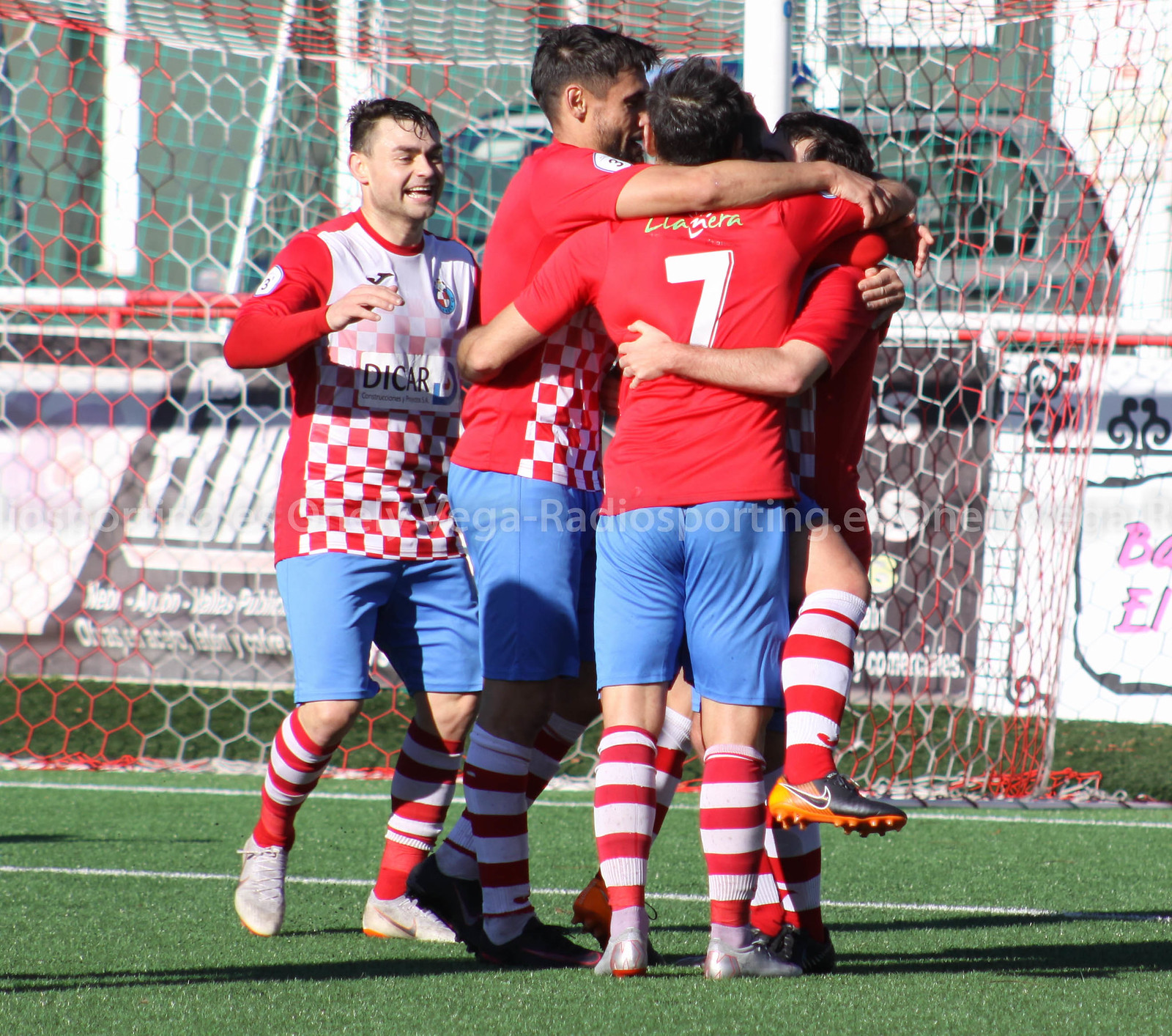The photograph captures a jubilant moment on a professional soccer field, where a group of soccer players are celebrating a likely victory through an emotional group hug. The field is meticulously maintained with fake green grass, marked by white lines delineating areas of play. Prominently visible in the background is a black, white, and red goal net, set against railing adorned with partially hidden, multicolored banners.

The players are uniformly dressed in distinctive outfits consisting of red short-sleeved t-shirts with white fronts, accented by a red and white checker pattern on the bottom half, accompanied by blue shorts and red socks with white horizontal stripes. Most of the players have dark hair, and among them, one player stands out facing away from the camera, displaying a large white number 7 on their back. Another player with short dark hair and a similar uniform, but with long sleeves, is running towards the group, smiling and possibly heading towards the goal. Their cleats vary slightly in color, with some sporting gray or silver and others dark with orange accents.

The scene radiates with shared happiness and excitement, encapsulated in the players' expressions and their united embrace.